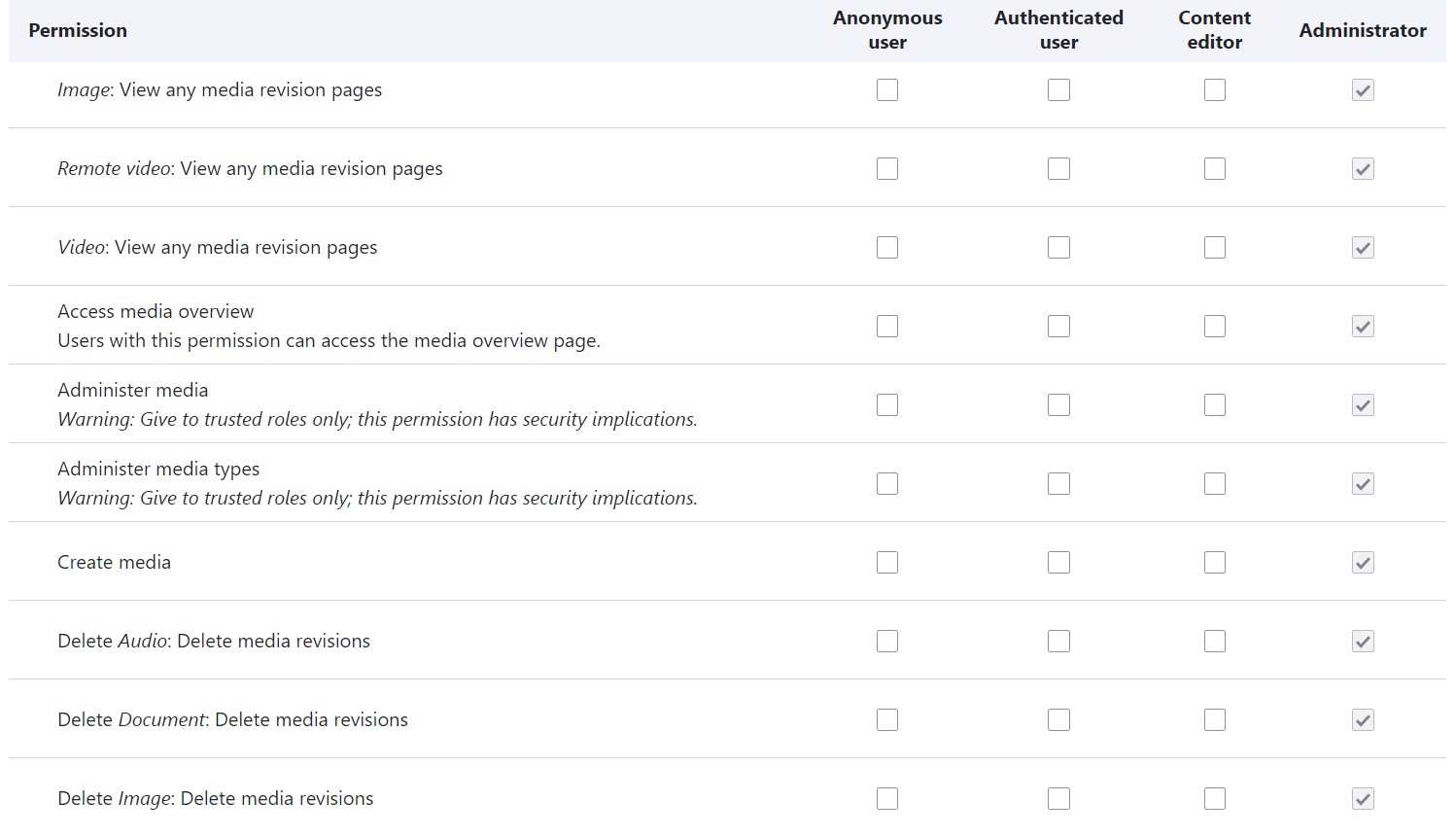The image, set against a white background, displays a detailed permissions matrix for different user roles within a content management system. The matrix includes roles such as 'Anonymous User,' 'Authenticated User,' 'Content Editor,' and 'Administrator.' Each role is associated with a series of permissions represented by checkboxes. 

For the 'Administrator' role, all the checkboxes are checked, indicating full permissions across various actions. These actions include 'Remote Video,' 'View Any Media,' 'Revision Pages,' 'Access Media Overview,' 'Administer Media,' and 'Administer Media Types.' Notably, several permissions like 'Administer Media' and 'Administer Media Types' are highlighted with a warning, suggesting that these should only be given to trusted roles due to their security implications. 

The comprehensive list for the 'Administrator' role also covers permissions to 'Create Media,' 'Delete Audio,' 'Delete Media Revisions,' 'Delete Document,' 'Delete Image,' among others. This layout emphasizes the extensive control and access granted to administrators in contrast to the more restricted permissions for other user roles.